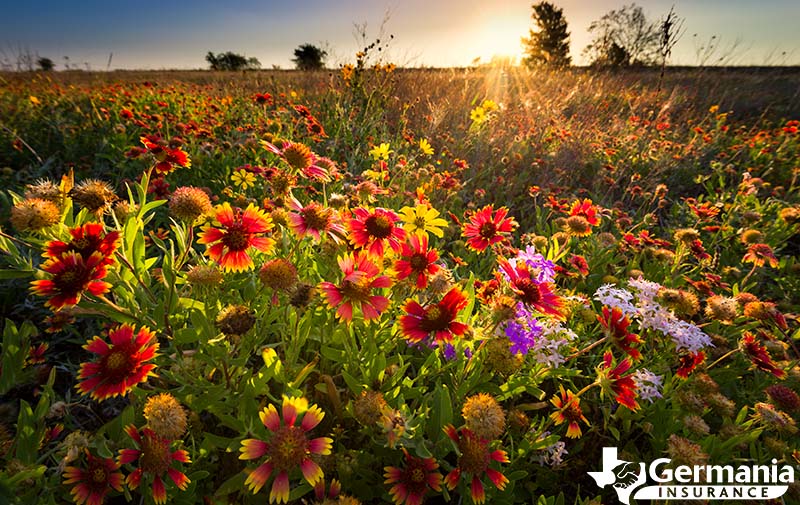The photograph captures a sprawling field of wildflowers bathed in the warm glow of sunset. The sun, with its radiant yellow glow, rests just above the horizon to the right of the center, casting a serene light over the entire scene. The sky transitions from a rich orange near the horizon to a deep blue at the top. The field itself is a vibrant tapestry of colors; predominantly, flowers with dark brown centers and red petals tipped in yellow dominate the scene, interspersed with lighter purple and pink blossoms. The flora, featuring long stems and green leaves, stretches out into the distance, gradually giving way to a hazy yellow grassland in the background. The farthest reaches of the field show sparse, fading clusters of flowers, enhancing the depth of the landscape. Small trees punctuate the distant horizon, adding to the natural charm of the scene. In the bottom right corner of the photograph, the logo of Germania Insurance—a depiction of the state of Texas with two hands shaking inside it—is prominently displayed, clearly marking the image as part of an advertisement.